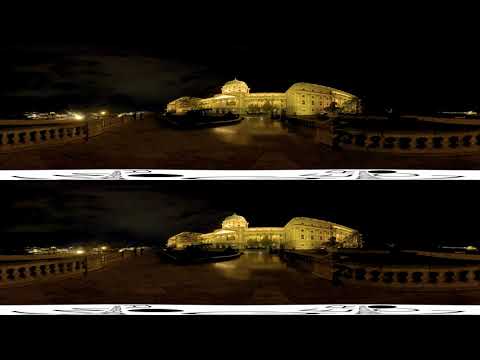The image displays two identical nighttime panoramic scenes, stacked one above the other with a thin white space separating them. It features a large, brightly lit, white building in the center, possibly a hotel, resort, or governmental villa with colonial architecture. The building spreads horizontally across the image, with four distinct vertical sections and a smaller, dome-shaped top in the center. A path leads up to the building from the front of the image, flanked by a fence made of cement pillars. The ground appears slightly shiny, reflecting the ambient light in the dark background.